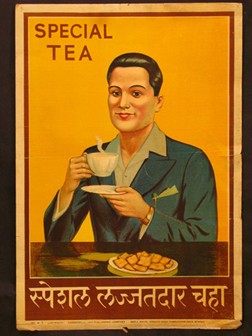In this richly detailed image, a well-dressed man with neatly coiffed, shiny dark hair is featured at the center, conveying a sense of contentment as he lightly stares ahead. He is elegantly attired in a brown suit layered over a green suit jacket with a light green shirt underneath. The man holds a white cup of tea with steam gently swirling upward in his right hand, while his left hand supports a matching white plate. Positioned in front of him is a brown table adorned with a plate of square, light brown biscuits.

The backdrop showcases a poster or package with the title "Special Tea" prominently printed in brown capitalized letters, encased in a rectangular shape. This title is accentuated with a maroon-colored border that adds to the visual appeal. The entire signage stands out against a striking gold background, and features gold-colored script at its base, which appears to be in an intricately styled, potentially Hindi font. Overall, the image exudes a warm and inviting allure, harmonizing the elegance of the man and the refined presentation of the tea.